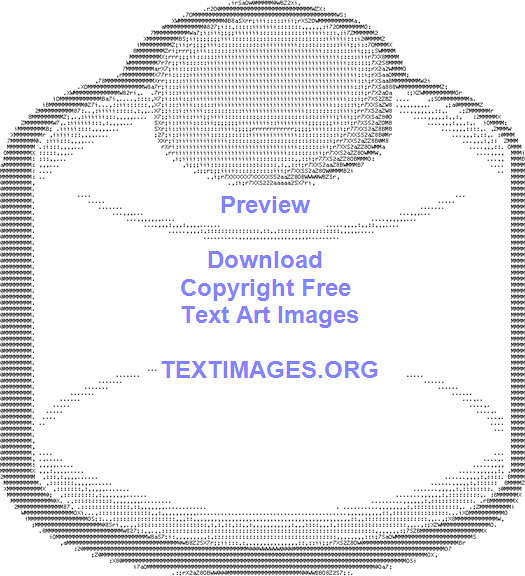This is a grayscale image composed entirely of text characters, designed to mimic the appearance of a small, clear bottle with a gray screw-on cap. The entire picture uses varying degrees of boldness and character placement to create shadows and definitions, giving it a pixelated, computer-generated look. The bottle's outline is detailed in dark text characters, enhancing the lid's shading and the overall shape. The background is stark white, providing contrast. Across the image, in blue text, it reads: "preview," "download," "copyright-free," "text art images," and in all caps, "TEXTIMAGES.ORG," indicating the source and nature of the image as a piece of computer-generated text art.